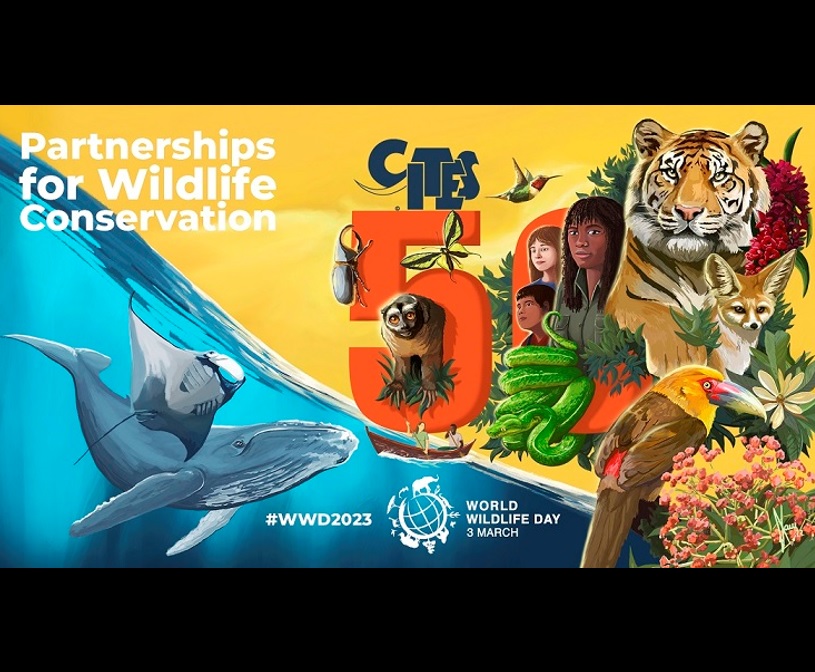A vibrant, animated promotional poster for World Wildlife Day 2023, featuring a harmonious blend of land and sea wildlife drawn in watercolor or acrylic style art. The poster is framed by thick black lines at the top and bottom, with a yellow background accentuated by a blue river flowing through the center. In the top left corner, the text "Partnerships for Wildlife Conservation" is prominently displayed in white font. Below this, the river contains detailed depictions of a large blue whale and a graceful stingray swimming. On the bottom portion of the river, "WWD 2023," accompanied by a globe symbol, is written in white text, followed by "World Wildlife Day 3 March."

On the right side, set against the yellow background, a rich tapestry of terrestrial animals is illustrated. This includes a light orange and black tiger, a white and brown fennec fox, and a brown and yellow bird perched above light red flowers. Additional creatures such as a monkey, a green snake, and vibrant bugs add to the scene's diversity. Three human figures, all facing to the left, contribute to the narrative of conservation partnerships - one with black hair and a green jacket, another with simply a face visible having black hair, and a third with long brown hair. This visually engaging poster captures the essence of global wildlife conservation efforts.